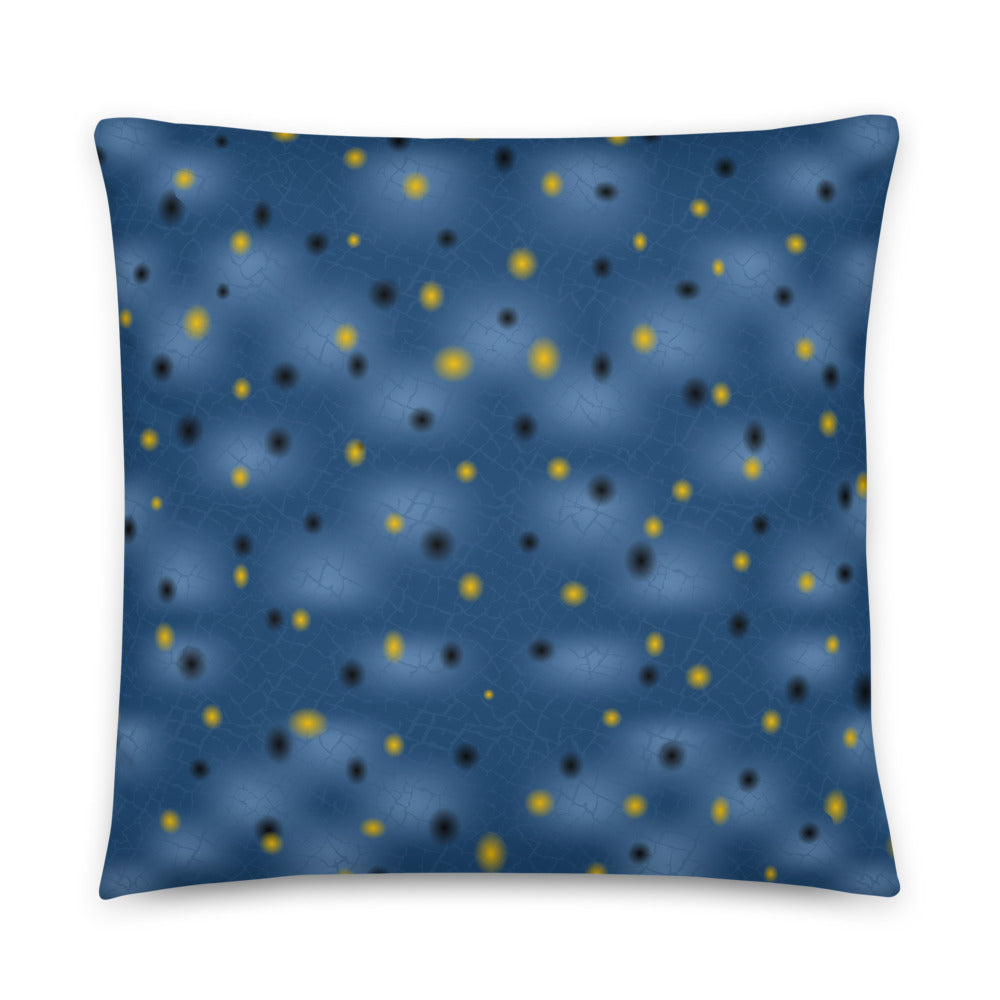The image depicts a predominantly blue pillow, possibly computer-generated, set against a white background. The pillow has a square shape with slightly rounded edges, giving it a soft, cushioned appearance. A striking pattern covers the pillow, featuring yellow and black dots interspersed with lighter blue spots. These dots and spots appear blurry in some areas, adding to the texture of the fabric. The pillow’s surface showcases visible threads and crack-like image details, particularly noticeable when zoomed in. The design seems to bulge slightly in the middle, likely due to the distribution of dots and the inherent softness of the material. The presence of shadowing under the pillow enhances its three-dimensional look, suggesting depth and making it seem almost like part of an avatar game.